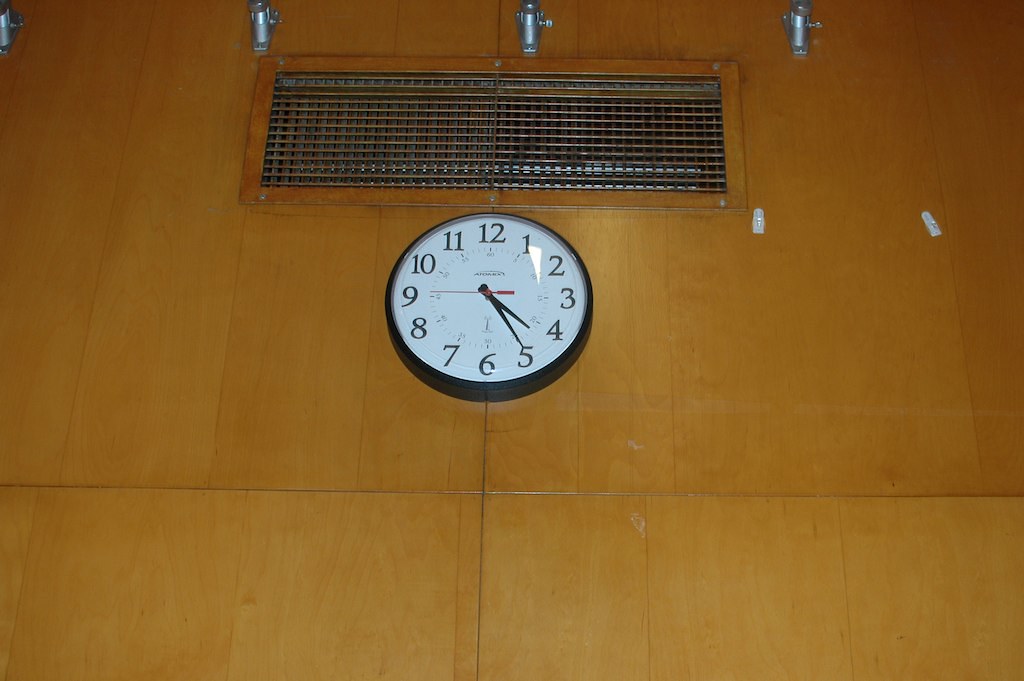The photograph captures an industrial interior setting, possibly within a business or educational institution, featuring a wall with warm, honey-colored wooden panels showcasing a prominent wood grain. Three unidentified silver objects protrude from the top of the wall, creating a point of curiosity. Below these objects is a silver metal grate, likely part of the heating or cooling system, bordered by a wooden frame matching the wall. To the right of the grate, two pieces of tape or similar materials are affixed. Positioned beneath the grate is a large, round clock with clearly marked numbers from 1 to 12, black hour and minute hands, and a distinctive red second hand.